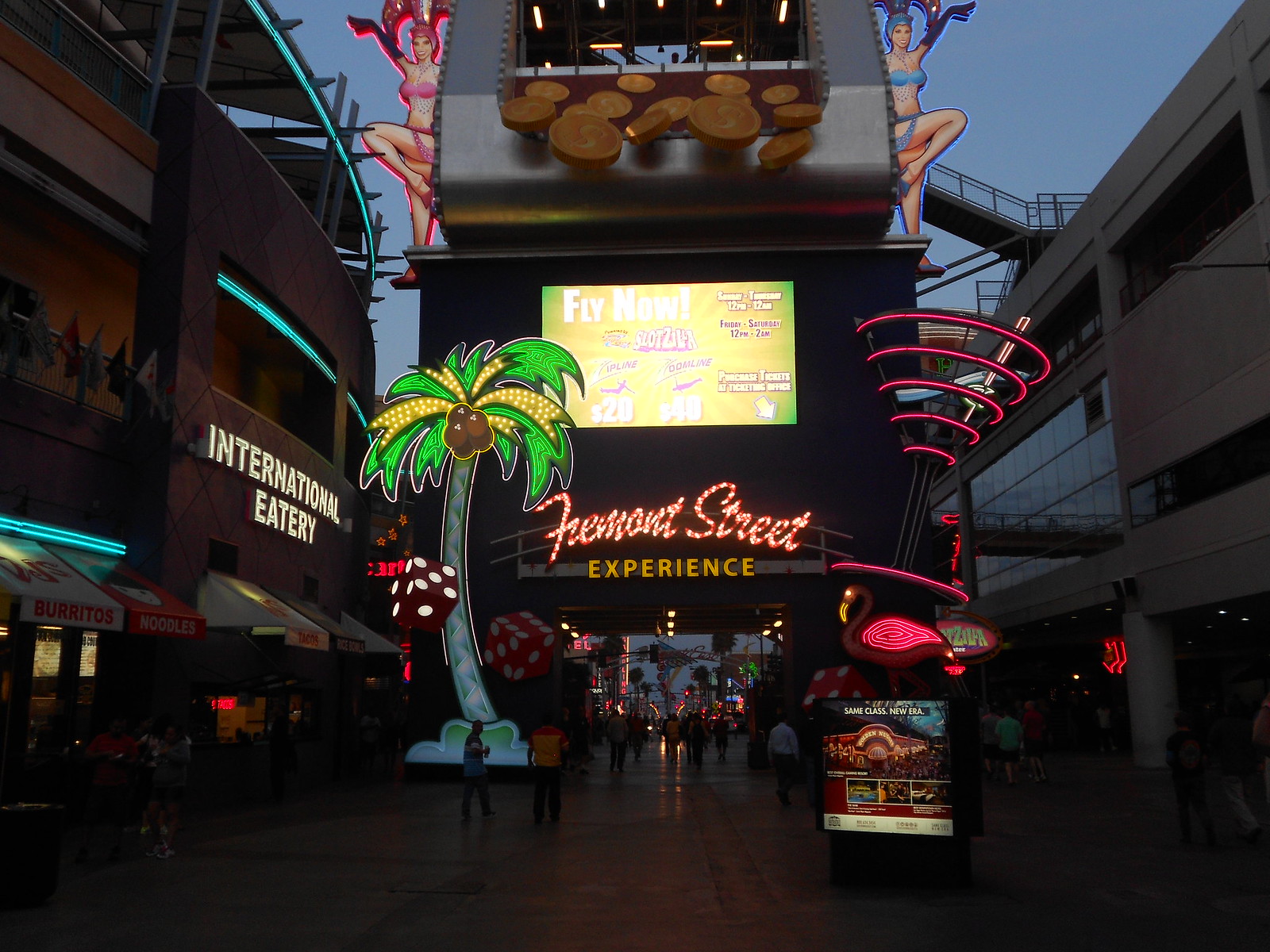The photograph captures an outdoor area of a bustling street arcade just before sunset. This rectangular image showcases the vibrant and lively Fremont Street Experience. Spanning the width of the image are two buildings on either side, connected overhead by an arched walkway emblazoned with the Fremont Street Experience sign. This sign serves as the centerpiece beneath a large, bright screen displaying various images, including coins falling and advertisements with scantily clad showgirls flanking each side.

To the left, a sign indicates the International Eatery, with various awnings below advertising burritos and noodles. The ground is dark, adding contrast to the surrounding illuminated elements. Prominently featured are an oversized glowing palm tree with coconuts and an equally large, bright pink martini glass. Additionally, there is a three-dimensional die, positioned beneath the International Eatery sign. 

Numerous light-up decorations, including a cube of dice and neon signs, enhance the festive atmosphere. In the middle area beneath the walkway, there are various people walking to and fro, emphasizing the area's extensive and lively nature. Above, the advertisement screen shows detailed promotions for nearby attractions and rides, with clear markers indicating times and ticket prices. The entire scene is framed by the open sky and further distant buildings, adding depth and showcasing the street's extensive scale and activity.